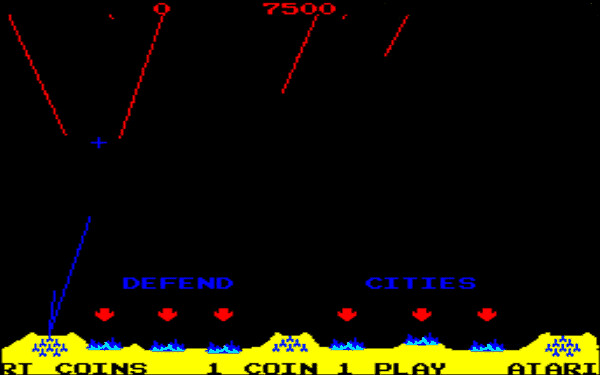Screen capture of an old Atari 8-bit video game. The screen background is predominantly black with various elements overlaying it. Red streaks ascend from the bottom and traverse diagonally across the screen, with one prominent streak starting from the upper left corner. At the very top center is the red score "7500". The bottom of the screen features a yellow terrain resembling a mountain range.

The lower part of the screen showcases several blue objects atop the yellow terrain. Specifically, there are six blue planes arranged symmetrically: three on the left and three on the right. Each of these planes is aligned beneath a red downward arrow, mirroring the planes' positions. These arrows are part of two separate groups with each group consisting of three arrows.

Above the groups of arrows, the phrase "DEFEND" in blue letters is positioned on the left while "CITIES" is displayed on the right. Additionally, there is a prominent blue cross near the middle left side of the screen, and a blue dotted line ascending from the bottom left corner.

At the bottom of the screen, it reads "RT coins, one coin, one play" and "Atari" is displayed in the bottom right corner.